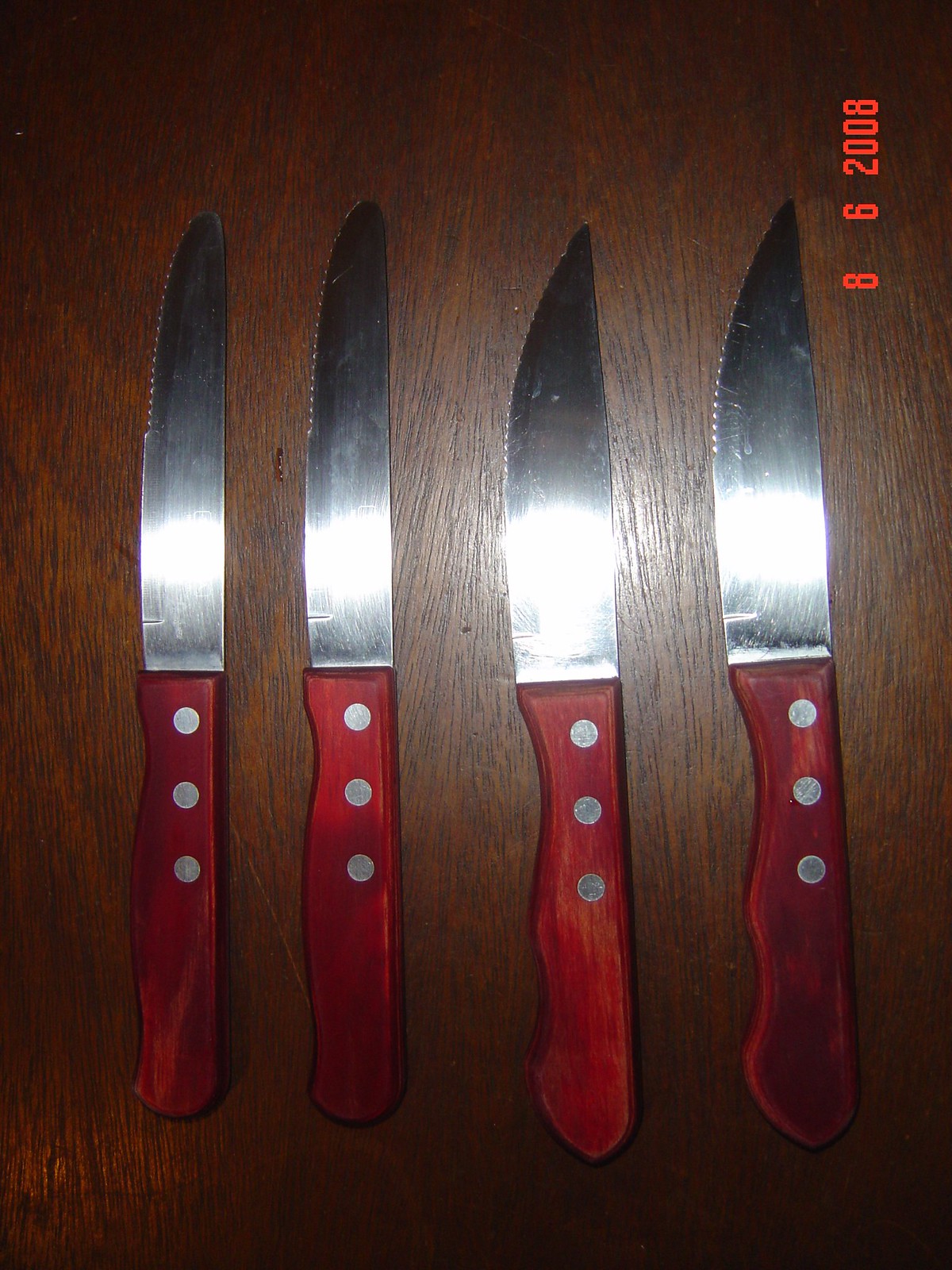This close-up color photograph, dated 8-6-2008 in orange text on the right-hand side, showcases a set of four knives laid out on a chocolate brown wooden table. The arrangement is orderly with the handles pointing downward and the blades facing to the left. All knives exhibit blades with a slightly serrated edge on the top half and reflect light, indicative of a flash used during the photograph. Each knife features a dark mahogany handle, secured by three silver rivets in a vertical line, and a shiny metal blade. The two knives on the left are butter knives with rounded tips, while the two on the right are slightly longer, broader, and have sharper, pointed tips. The handles of each knife are maroon-red stained wood with a distinctive grip that accommodates fingers comfortably, especially noticeable in the paring knives on the right. The harmonious yet distinct features of each knife suggest they are part of the same set.